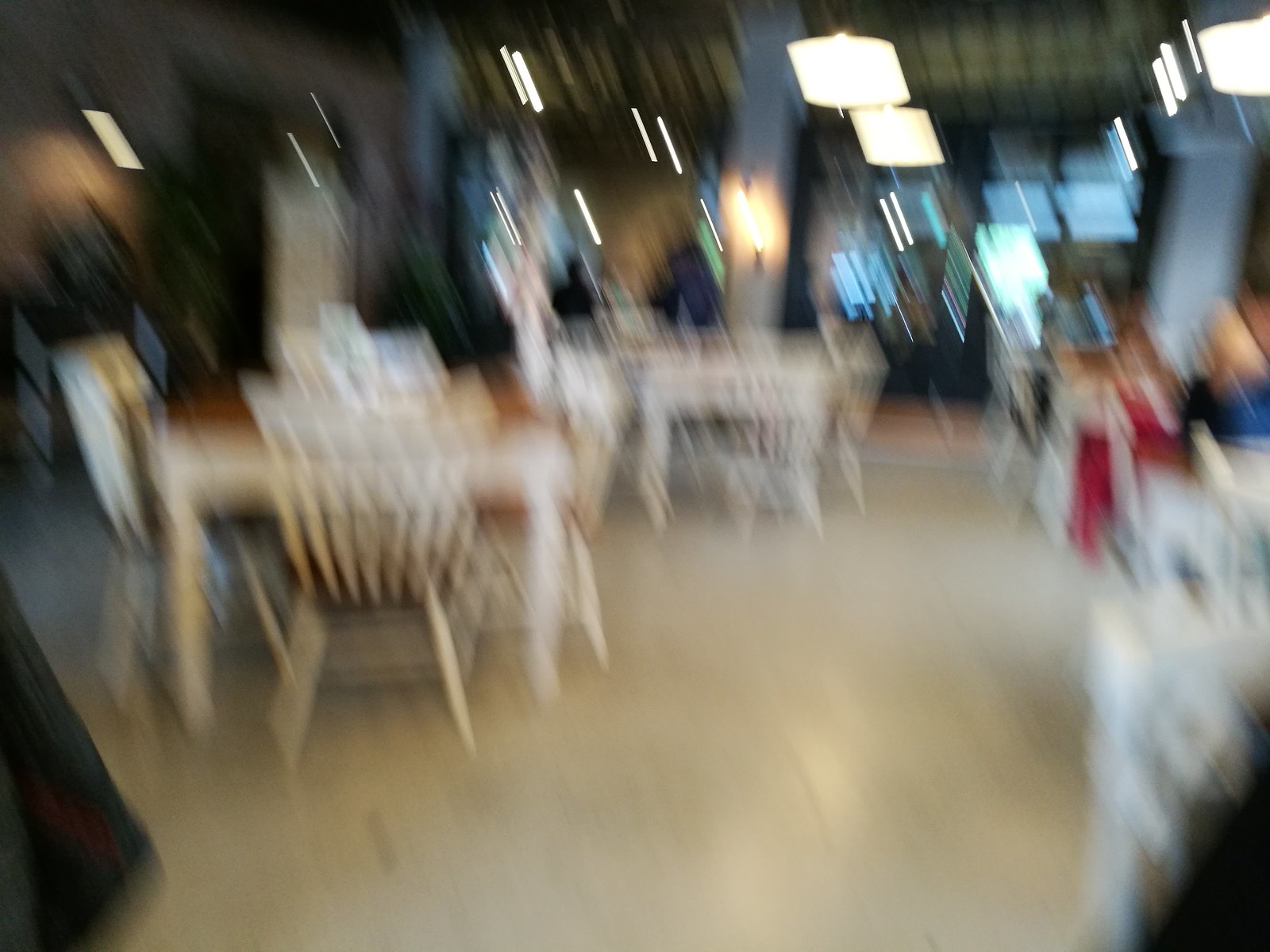The image depicts a dining hall or restaurant, albeit very blurry. The hall is furnished with several square tables featuring brown wooden tops and four white legs. Each table is accompanied by four chairs, one on each side, creating a cohesive set with the seats mirroring the table tops' wooden finish while the legs and backs of the chairs remain white. The floor is covered in white tile. The room is well-lit by overhead lighting, and in the background, there appear to be windows, possibly indicating an entrance or exit. No one is seated at the tables, and all the chairs are neatly pushed in, suggesting the area is either prepared in anticipation of guests or has recently been vacated.